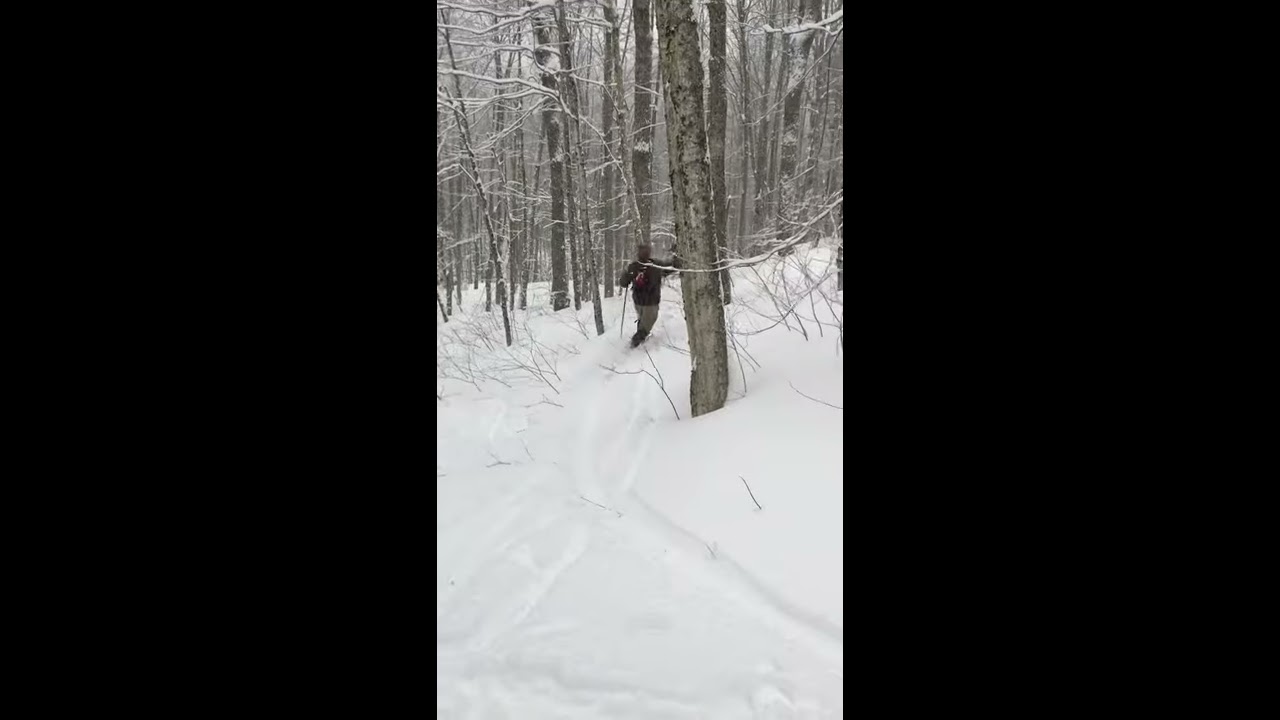In this photograph, a person is trekking through a snowy, barren forest. The image is framed in a vertical aspect, with thick black bars on both sides, as if captured on a cell phone. The forest, shrouded in winter's grasp, features trees stripped of leaves, their grayish-brown bark contrasting starkly against the white snow. Between the trees, smaller limbs and twigs poke out from the snow-covered ground. 

In the distance, partially obscured by a large snow-covered tree, the person is visible, clad in a dark coat and gray pants. They appear to be engaged in cross-country skiing, gripping ski poles in both hands, though the skis themselves are buried in the deep snow. A winding trail of tracks leads from their position, splitting and converging at various points, hinting at either multiple routes they have taken or previous travelers along the same path. The overall scene is a monochrome blend of white and muted browns and grays, emphasizing the stark, chilly solitude of the winter landscape.